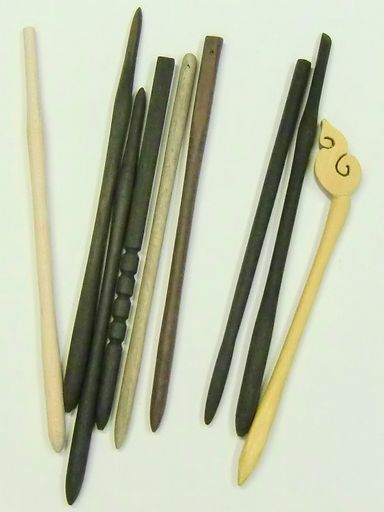The image depicts an assortment of nine wooden implements arranged vertically against a flat, light gray background. Each implement is long, thin, and cylindrical, resembling the shape of a pencil, toothpick, or stylus, with one end pointed and many featuring a small hole punched near the top. The implements vary in color and finish, ranging from very light, unfinished wood to dark, polished wood, with one showcasing a greenish-brown hue. The sequence of the implements starts with a tan one on the far left, followed by three black ones, a darker brown with a carved ornament resembling a seashell or flame at the top, two more black ones, and finally another tan implement with a decorative, swirly S-shaped carving at the top. Additionally, one of the lighter implements has a series of carvings in the middle that resembles a row of beads. The overall arrangement and intricate details of the carvings add a unique visual interest to the assortment.